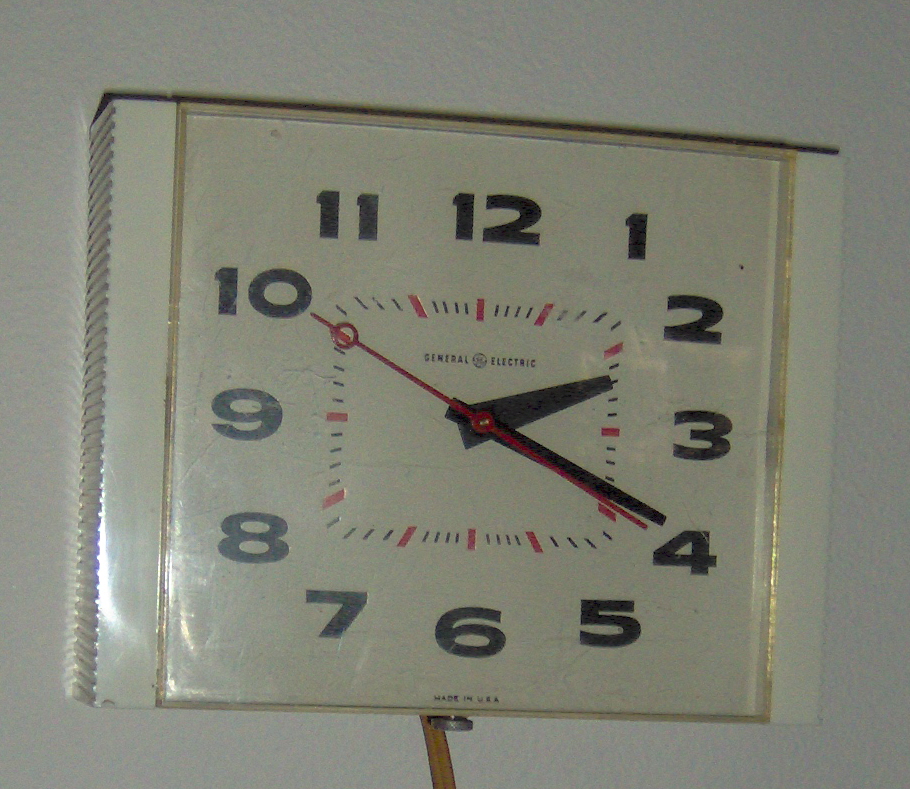The image features a vintage, square-shaped clock made by General Electric, with a distinctly older, sturdy build. The clock, displaying the time as 2:19, features bold black numbers 1 through 12 arranged in a typical circular format, with smaller black markers for each minute and additional red markers for every five minutes. The hour and minute hands are black, while the second hand is red with a small circle at its tip. Below the number 6, the text reads "Made in USA." The clock face is covered by a clear plastic or glass surface, which has a subtle light brown tint. The edges of the clock have white, uneven grooves reminiscent of ruffled chips. There is a metal screw and a brown cable emerging from the bottom of the clock. The clock is centered against a white background, mounted on a textured wall.